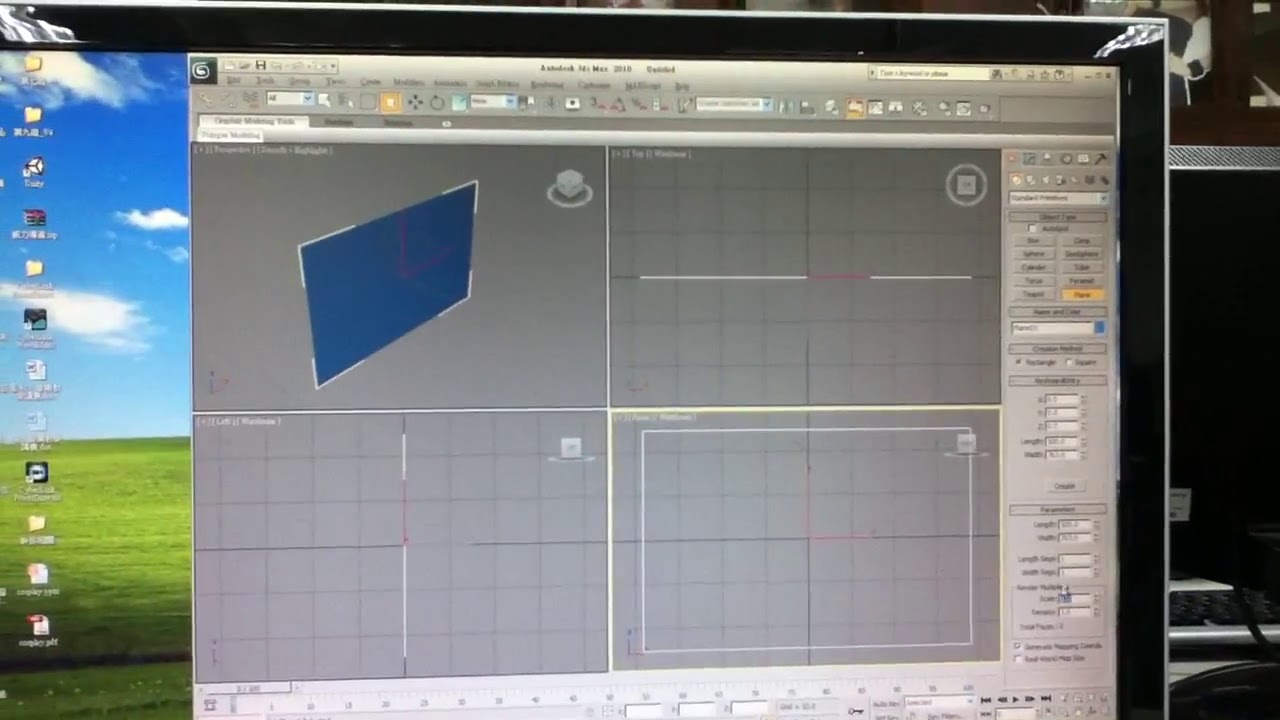The image shows an LCD monitor with a black bezel, displaying a Windows operating system desktop. The majority of the screen is occupied by a complex application that resembles a 3D drawing or CAD software, possibly similar to AutoCAD. The software interface is cluttered with numerous buttons and technical terms, and it is divided into four distinct panes in a grid layout. The top-left pane shows a blue-colored 2D plane, suggesting the modeling of a flat rectangle, while the other panes display outlines from different camera angles.

On the left side of the monitor, which takes up about 10% of the screen, the classic Windows grassy hill wallpaper with a blue sky and white clouds is visible, along with several desktop icons indicating a PDF file, several folders, and possibly a Microsoft Word document. The monitor is positioned on a desk, and some elements of the workspace can be seen, including the back of another monitor and a keyboard.